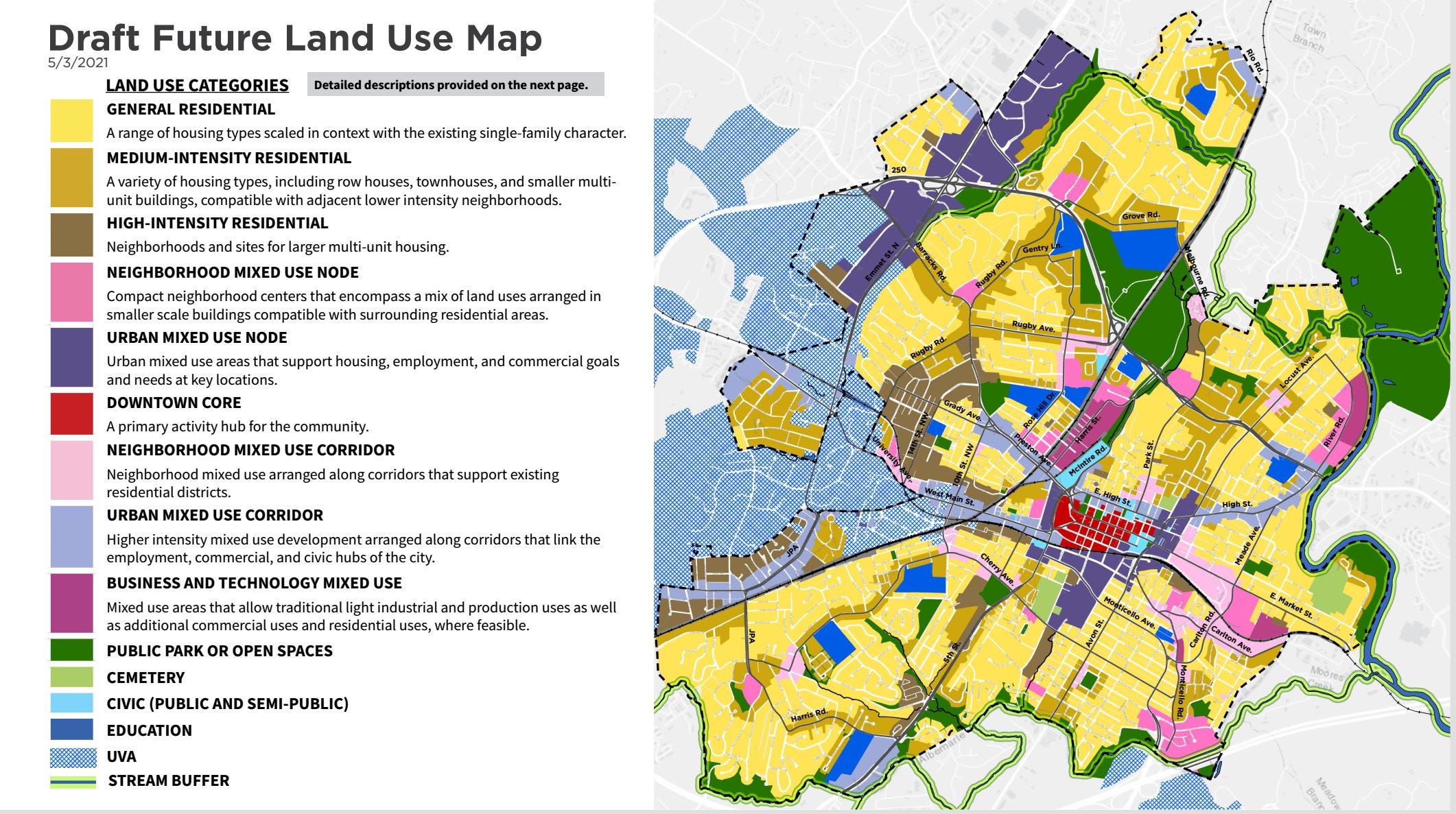This image is a highly detailed, illustrated aerial map labeled "Draft Future Land Use Map," dated either May 3rd or May 5th, 2021. The map provides a comprehensive overview of the cityscape, showcasing various neighborhoods and zones through a vibrant array of approximately 20 different colors. The colors represent distinct land use categories, with yellow being the most predominant, indicating general residential areas. Other notable colors include dark red for the downtown core, described as the primary activity hub for the community, and green for public parks or open spaces. The left side of the map features a key that breaks down these colors and their meanings, including medium and high-intensity residential, urban mixed-use nodes, neighborhoods, urban business areas, cemeteries, civic centers, and educational facilities. This map is intended to outline the future land use plans of the city, detailing how different sections will be purposed, potentially indicating city expansion and development strategies.